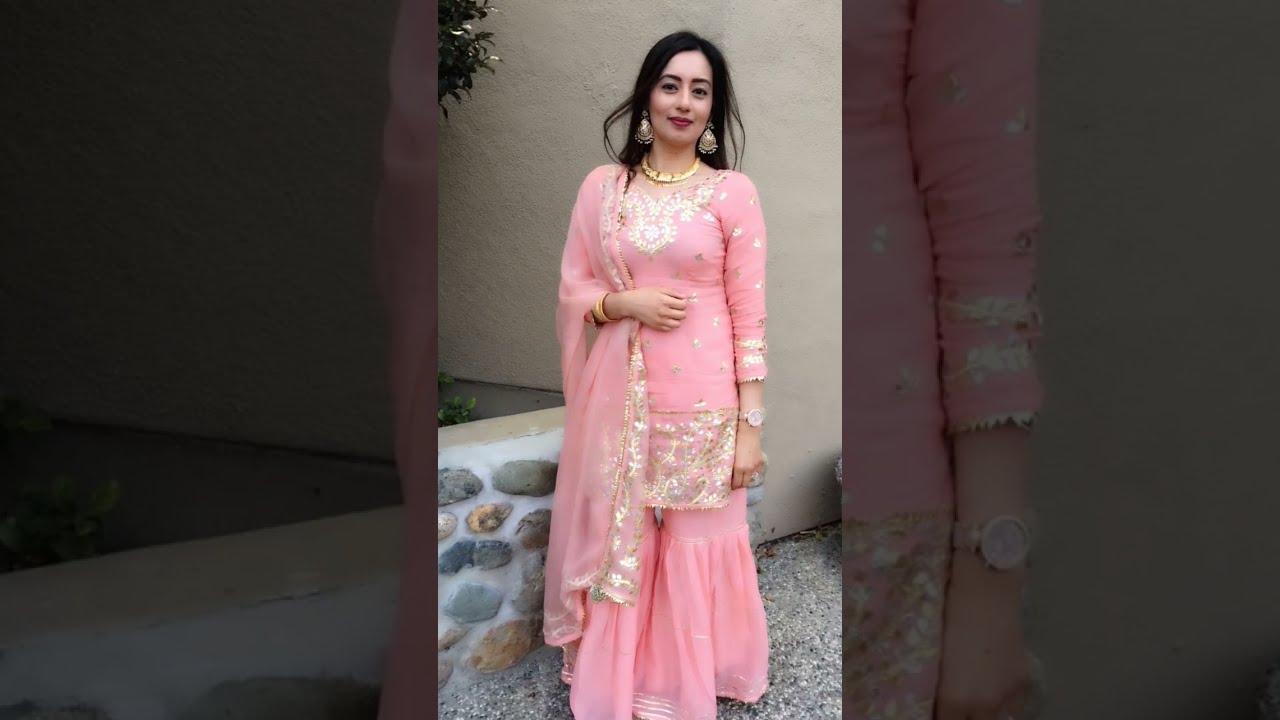The photograph features an attractive young woman with a light skin complexion and long, flowing dark hair. She appears to be of Indian, South Asian, or potentially Middle Eastern descent. The woman is elegantly dressed in a vibrant pink dress adorned with white lace edging and gold accents, which contributes to a flouncy and festive appearance. Draped over her right shoulder is a luxurious sari-type cape with silver detailing. Her accessories include a white beaded necklace, large gold drop earrings, and a silver wristwatch on her left wrist. She gazes directly into the camera with her right arm bent at the elbow, hand positioned in front of her midriff, while her left arm hangs relaxed by her side. The image, taken outdoors in daylight, reveals a white wall and a stone half-wall or railing from the hips down, further enriching the setting's natural light and serene ambiance.